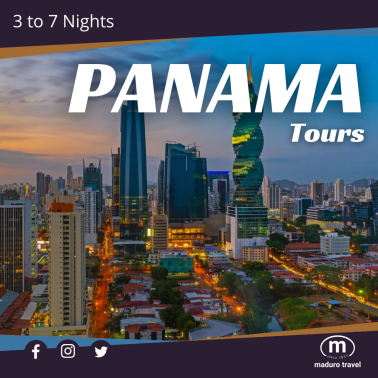Considering a vacation in Panama? This image captures a promotional banner for Panama, highlighting a dreamy travel experience. Dominated by the text "Panama" in large white letters, the word "Tours" appears smaller underneath the "MA" to the right. The scene features a mesmerizing view of Panama City's downtown at dusk, showcasing a blend of modern skyscrapers and historic buildings. Two prominent skyscrapers catch the eye—one with a unique spiral design and reflective glass windows, seemingly glowing as the sunlight hits it. Between them, a smaller structure adds to the urban charm.

The cityscape is lively with bustling traffic, as indicated by visible car headlights and brake lights. The sky transitions from blue to shades of pink, enhancing the picturesque ambiance. A purple banner at the top left corner announces "Three to Seven Nights" in white text, gradually narrowing towards the right. Social media icons for Facebook, Instagram, and Twitter are displayed on the left, directing visitors to Maduro Travel's social media profiles, indicated by an "M" emblem on the far right.

While the specifics of the travel package, such as costs or contact information, are not provided, the scene effectively sells Panama as a destination. The distant horizon hints at the ocean, shrouded slightly in fog, adding to the allure of this vibrant cityscape.